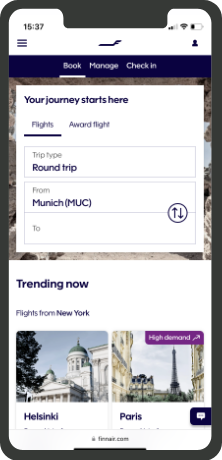An image of a smartphone and a tablet, both displaying a flight booking application, is shown. The smartphone, in full Wi-Fi mode but with a partially depleted battery, exhibits a user interface with an orange banner reading "Your Journey Starts Here," set against a backdrop comprised of rugged rock formations. The layout features various travel options like "Award Flight" and "Round Trip" for routes originating from Munich. Dropping down with an arrow icon, the focus then shifts to a 'Check-in/Manage Booking' window. 

In the background, there are white text panels listing trending flights: a New York flight labeled against a stark white background and another, presumably heading to Helsinki, characterized by a blue backdrop depicting prominent buildings. To the right, there's an iconic representation of the Eiffel Tower, set beneath a cloudy sky and surrounded by slender black high-rises, all cast in a purple hue. The webpage is branded "finnair.com," with darkened, possibly vignetted, edges around the screen, emphasizing the immersive experience offered by the travel app.